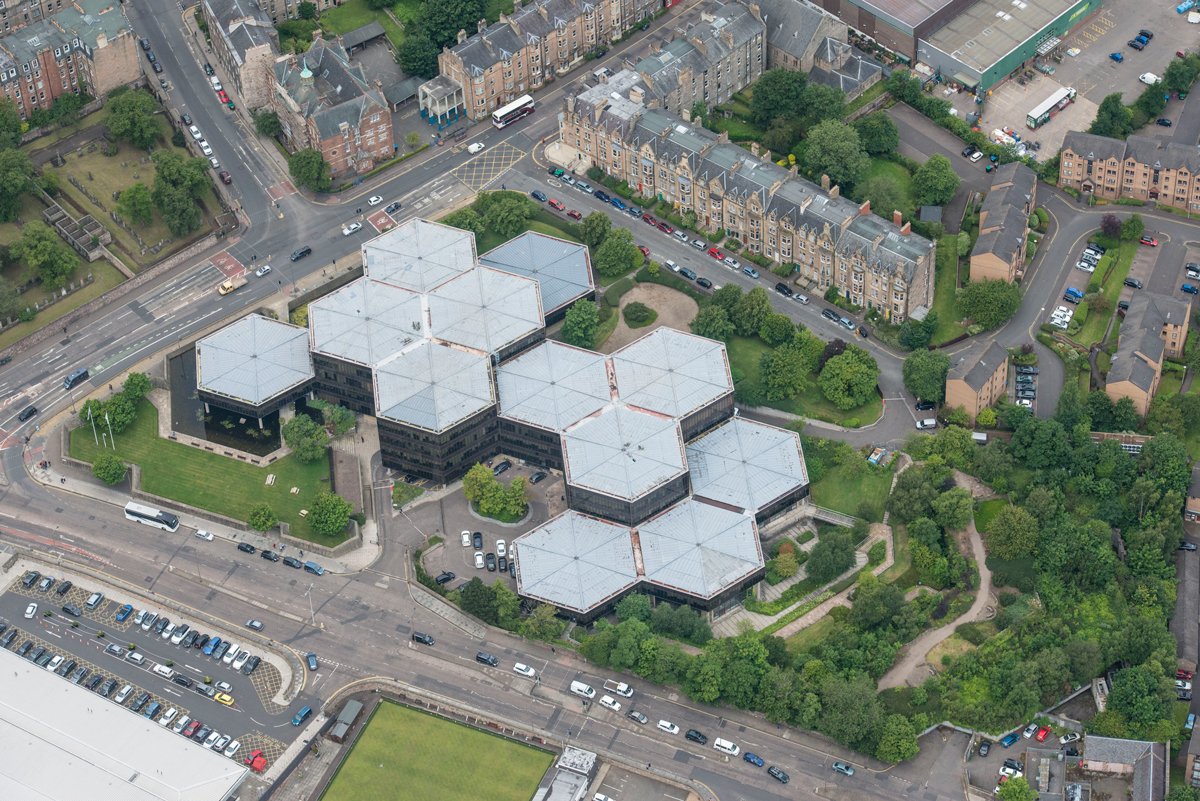This aerial photograph captures a highly distinctive complex of interconnected, hexagon-shaped buildings featuring white rooftops and black and gray facades. These hexagonal structures, numbering between 10 to 12, vary in height from one to six stories, with the tallest ones located centrally, near what appears to be a main entrance. The surrounding landscape features lush green trees and patches of grass, providing a vibrant contrast to the geometric layout of the buildings. In the vicinity, there are additional historic brick and stone buildings in shades of gray, red, and brown, along with a mix of homes and businesses. The area is bisected by gray streets and dotted with a variety of multicolored cars, including black, white, gray, red, yellow, and blue, as well as a visible bus and semi-trailer. This idyllic scene, devoid of any visible people or text, portrays an organized and possibly institutional setting that could be part of a college campus or an industrial office complex.